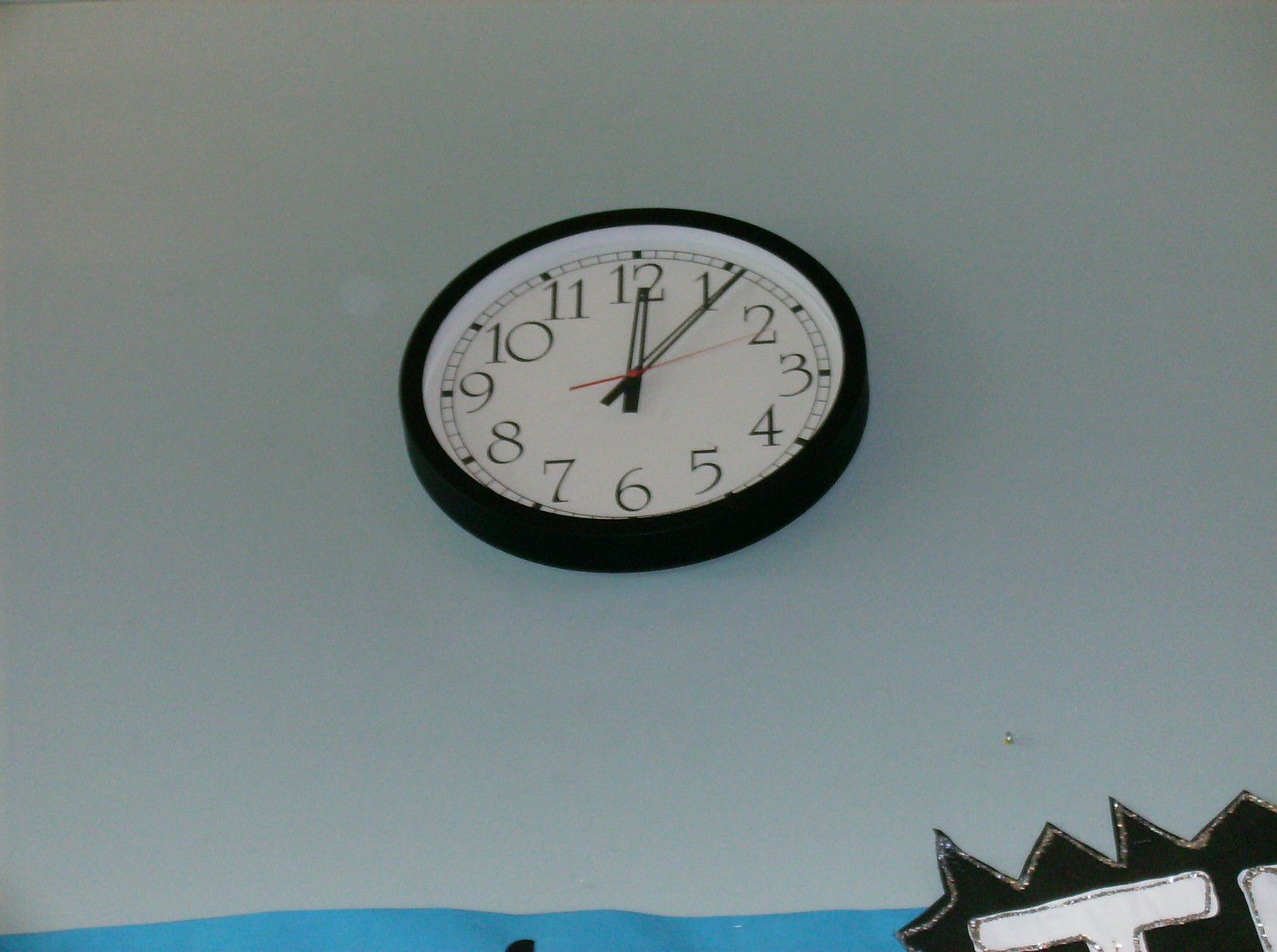The image shows a close-up, angled view of an analog clock hanging on what appears to be a light-colored wall. The clock has a stark white face with large, clear numbers in a simple, bold font—definitely not Roman numerals—encircled by black minute markers, with every fifth minute indicated by a slightly thicker line. The time reads 12:06, as the hour hand points to the 12 and the minute hand, with a distinct cutout making it hollow in the middle, is slightly past the 1. The clock has a thick, black rim around its edge, adding to its prominence on the wall. In the bottom right corner of the photograph, there's a partial view of a decorative element—a poster board cutout or sign—that features the top part of a white letter "T," edged with silver glitter. Additionally, at the bottom edge of the image, a blue banner appears, detailed with wavy patterns and accompanied by a small glimpse of a black marker. The overall scene also includes the suggestion of an industrial aesthetic, underscored by the sparse wall and functional design of the clock.